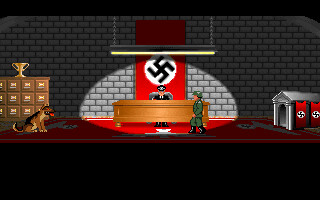The image appears to be a pixelated, flash-style still from a video game, depicting a Nazi-themed setting. Centrally located is a large wooden desk, occupied by a figure resembling Hitler, who is seated and wearing a black hat. Behind him hangs a prominent red flag featuring a black swastika in a white circle, set against a backdrop of silver brick walls. A bright light or spotlight is focused on the desk and a soldier dressed in a green uniform, green hat, and black boots, who is walking to the left in front of the desk. To the left side of the image is a German Shepherd dog, sitting with its pink tongue visible, in front of wooden filing cabinets that have a gold trophy placed on top. On the right side of the image, there’s a small structure, possibly a doghouse, adorned with two red banners, each also displaying a swastika.